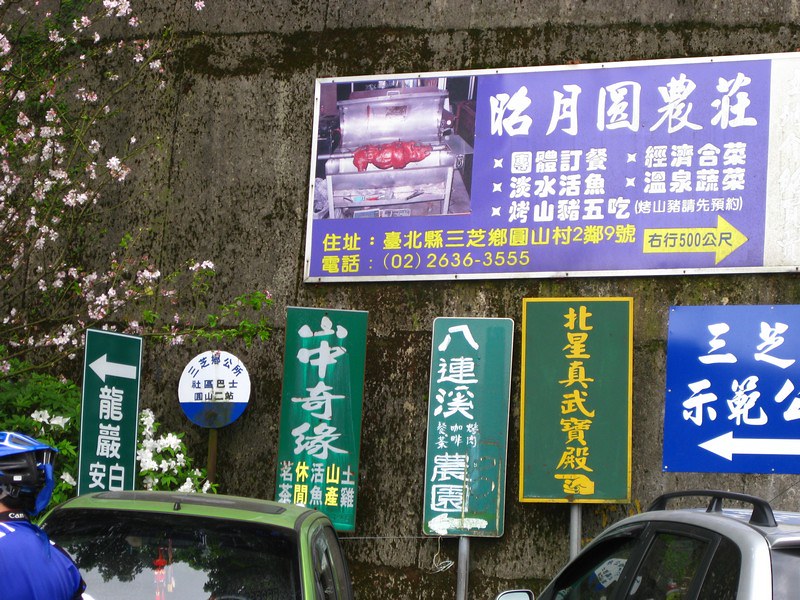In this image, we see a large, old gray brick wall adorned with an array of road and directional signs, prominently featuring kanji, indicating that this scene is likely set in either China or Japan. The most notable sign at the top of the image is a large, unusual information sign with foreign text that includes numbers like 02 and 26-36-3555. Several of the signs are mounted on individual metal poles, while others hang directly from the wall. The bottom corners of the image reveal a cyclist wearing a helmet in the bottom left, suggesting proximity to a cycling area, and a few cars parked in the bottom right and left areas. The overall scene gives a distinct impression of a bustling area with significant informational signage.